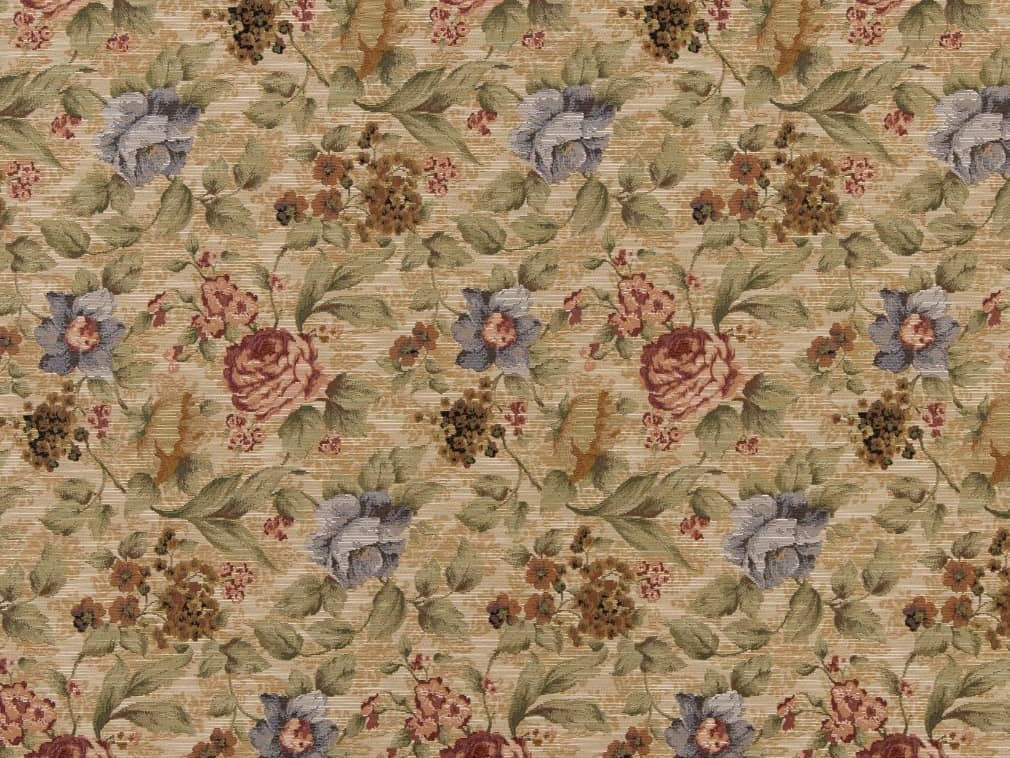The image is a close-up of what seems to be a textile, possibly wallpaper, adorned with a detailed floral pattern. The background is a muted pale beige, faintly brocaded, adding texture and depth to the composition. The primary floral elements include red carnations and another blue flower, both depicted with intricate petals and accompanied by various green leaves and occasional stems. Additionally, smaller clustered flowers in a dark orange, almost brown hue, and light brown blooms intermingle with the main flowers. The color palette is limited yet harmonious, featuring muted tones of blues, greens, browns, and occasional salmon-pink tints that contribute to a slightly dated, vintage aura. Overall, the pattern is dense and noisy, suggesting it might be used for an ornate sofa or traditional wallpaper, characterized by its repetitive and textured design.